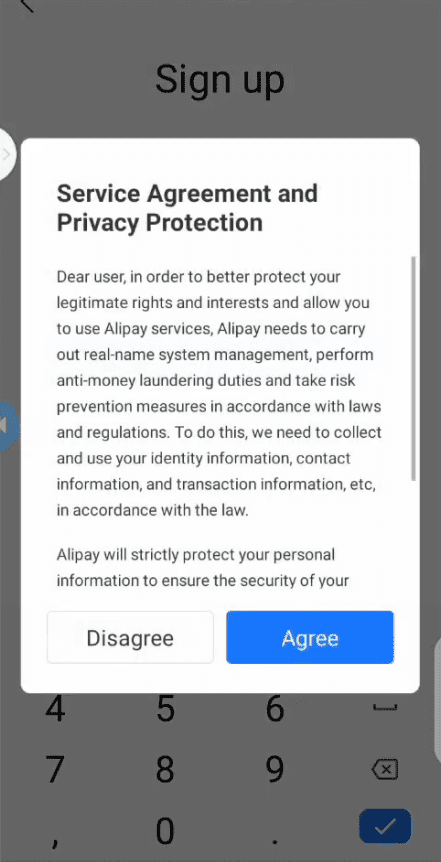This image is a detailed screenshot of a sign-up page for Alipay, presenting the user with the Service Agreement and Privacy Protection policies. At the top, there's an inviting heading, "Dear User." The text emphasizes the necessity for Alipay to collect and use the user’s identity, contact, and transaction information to comply with legal requirements such as real-name system management, anti-money laundering duties, and risk prevention measures. The message assures users that Alipay will strictly protect their personal information to ensure its security. The full text of the agreement requires scrolling to view. Toward the bottom of the screen, there are prominent options to either "Agree" or "Disagree" with the terms. The entire image is encapsulated within a rectangular frame, with no other significant elements present.